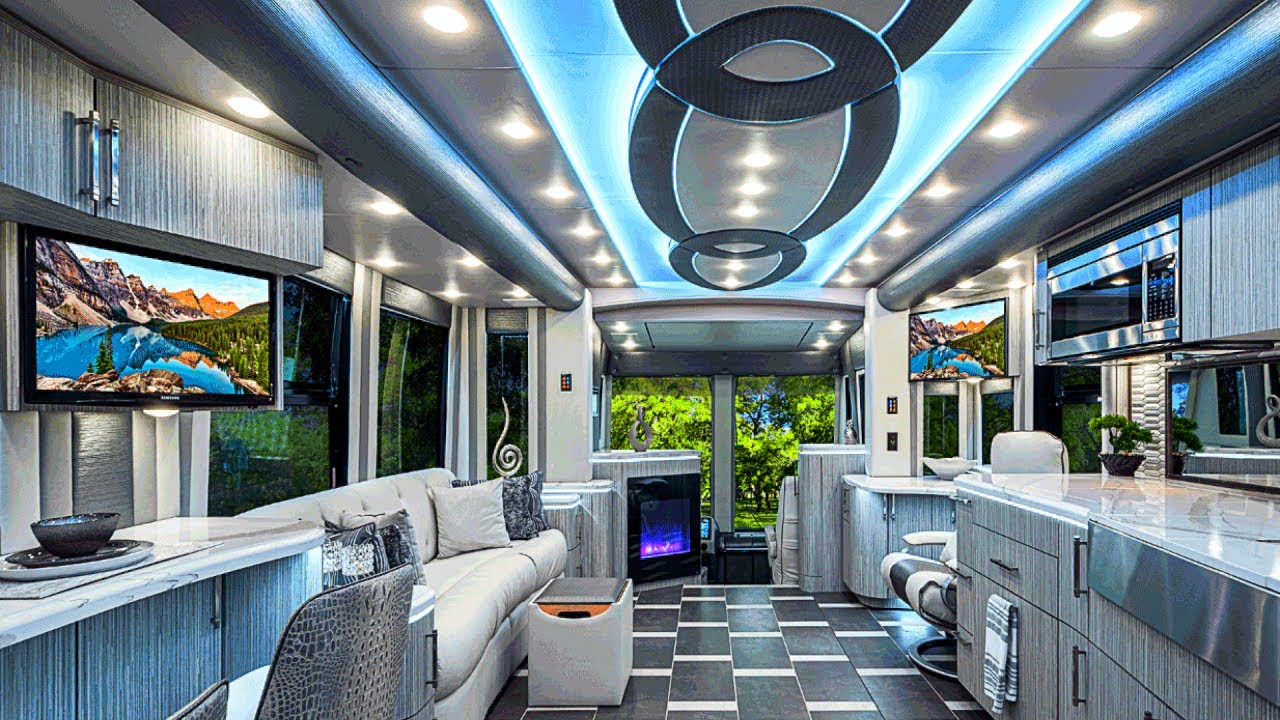This image depicts the interior of a stylish and modern RV or tiny home with a sophisticated feel. The space is narrow but appears elongated, filled with numerous windows on every side, providing ample natural light and a view of lush greenery outside. The decor throughout is sleek, with a contemporary gray and white palette. The ceiling features intricate designs with blue stripes and circular patterns, complementing the array of lights that are both white and blue. 

On the left side, there is a white couch situated under more windows, a counter with associated cabinets, and a TV mounted to the wall. The gray and white tile flooring enhances the modern ambiance. The right side of the room includes another TV mounted on the wall, a chair, and a well-equipped kitchen area with silver shelving, a microwave, a stove, and ample counter space. A bar-type counter offers seating for one, with a set plate and bowl placed neatly on top. The overall look is polished and seems almost computer-generated due to its high level of cleanliness and shine. At the far end, presumably, there is another large window which could potentially be a fireplace positioned nearby.